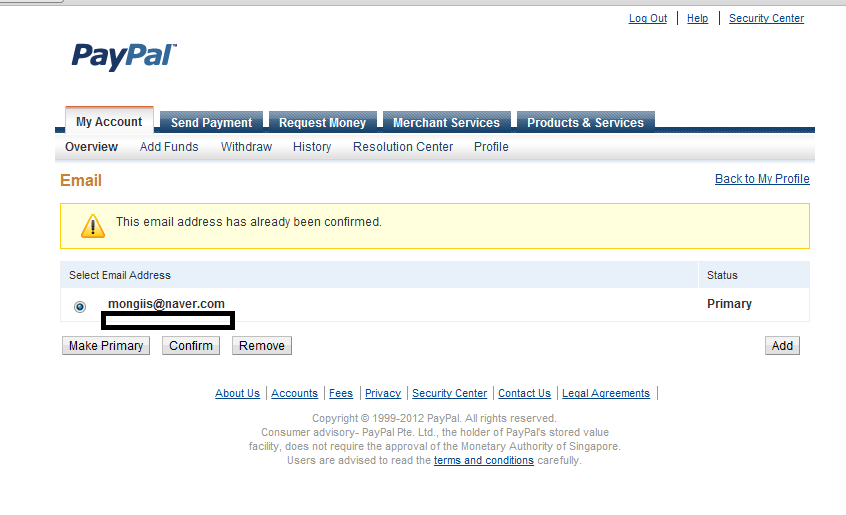This detailed screenshot captures an old PayPal account interface, distinctly marked by its outdated layout. The top left corner showcases the dark blue PayPal logo, while the top right corner features options like "Log Out," "Help," and "Security Center." Prominent menu tabs at the top include "My Account," "Send Payment," "Request Payment," "Merchant Services," and "Product Displays." Within the "My Account" tab, there are sub-menu options like "Overview," "Add Funds," "Withdraw," "History," "Resolution Center," and "Profile." The focal point of this screenshot is the email management section, identified by a header with "Email" and a link labeled "Back to Profile." A notable yellow alert box with exclamation points indicates that "this email address has already been confirmed." Below this, there's instruction to "Select Email Address," displaying one email: "mongis@neighbor.com" marked as 'Primary.' Functional buttons beside it allow actions such as "Make Primary," "Confirm," "Remove," and "Add." The page footer contains standard PayPal information, including links to "About Us," "Accounts," "Fees," "Privacy," "Security Center," "Contact Us," "Legal Agreements," and copyright details ranging from 1999 to a possible typo of "2020-2012," along with a reference to terms regulated by the Monetary Authority of Singapore.